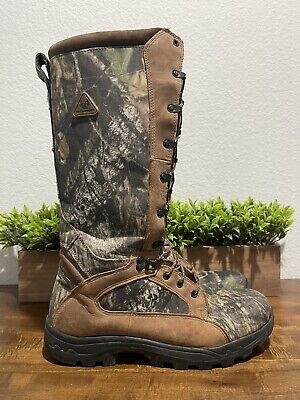This image features a pair of sturdy, camouflage-printed boots with a brown suede trim and black grommets for the laces. The boots are mid-calf height and sport thick, black rubber soles with prominent tread, suggesting durability and ruggedness. The camouflage pattern, in shades of green, grey, black, and white, appears on the main body of the boots, blending seamlessly with natural surroundings. Brown suede trims run along the top edges and from the top of the boot to the toe area, where thin brown trimmings accent the design.

The boots are positioned on a wooden floor with prominent dark brown grain, hinting at a rustic or outdoor setting. Behind the boots, a rectangular wooden planter is visible, filled with greenery or low-level plants, and it rests against a light-colored, textured wall, possibly stucco or cream-grey in color. There is a faint indication of a toe of the second boot in the background, confirming it is indeed a pair. The overall setting gives the impression of a blend between rugged outdoor utility and a stylized, natural aesthetic.